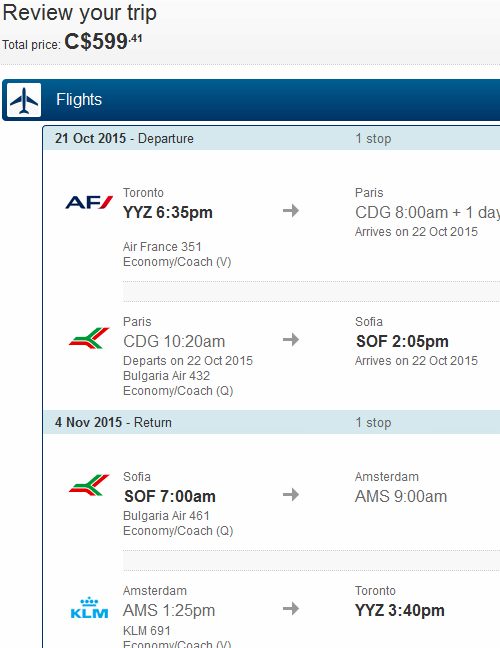The image depicts the "Review Your Trip" section of a flight booking app or website. At the top, there is a gray-colored box displaying the total cost of the trip, which is $599.41. Next to the total amount, there are currency symbols "C" and "$" on the left side.

Below this, a blue box is prominently featured. On the left side of the blue box, there is an icon of a white square with a blue airplane inside. Adjacent to the icon, the word "Flights" is written in white text.

Underneath the blue box, there is additional detailed information divided into different sections. The first section reveals the departure details, stating "21 October 2015" as the departure date, and mentions "one stop" on the right. The section is introduced with a logo "FJ" and a tricolor logo in white, red, and green. The flight route is from "Toronto to Paris" followed by "Paris to Sofia."

The second section specifies the return details, marked with "4th of November 2015" as the return date with "one stop." The return flight is from "Sofia to Amsterdam," and then "Amsterdam to Toronto," serviced by KLM airlines.